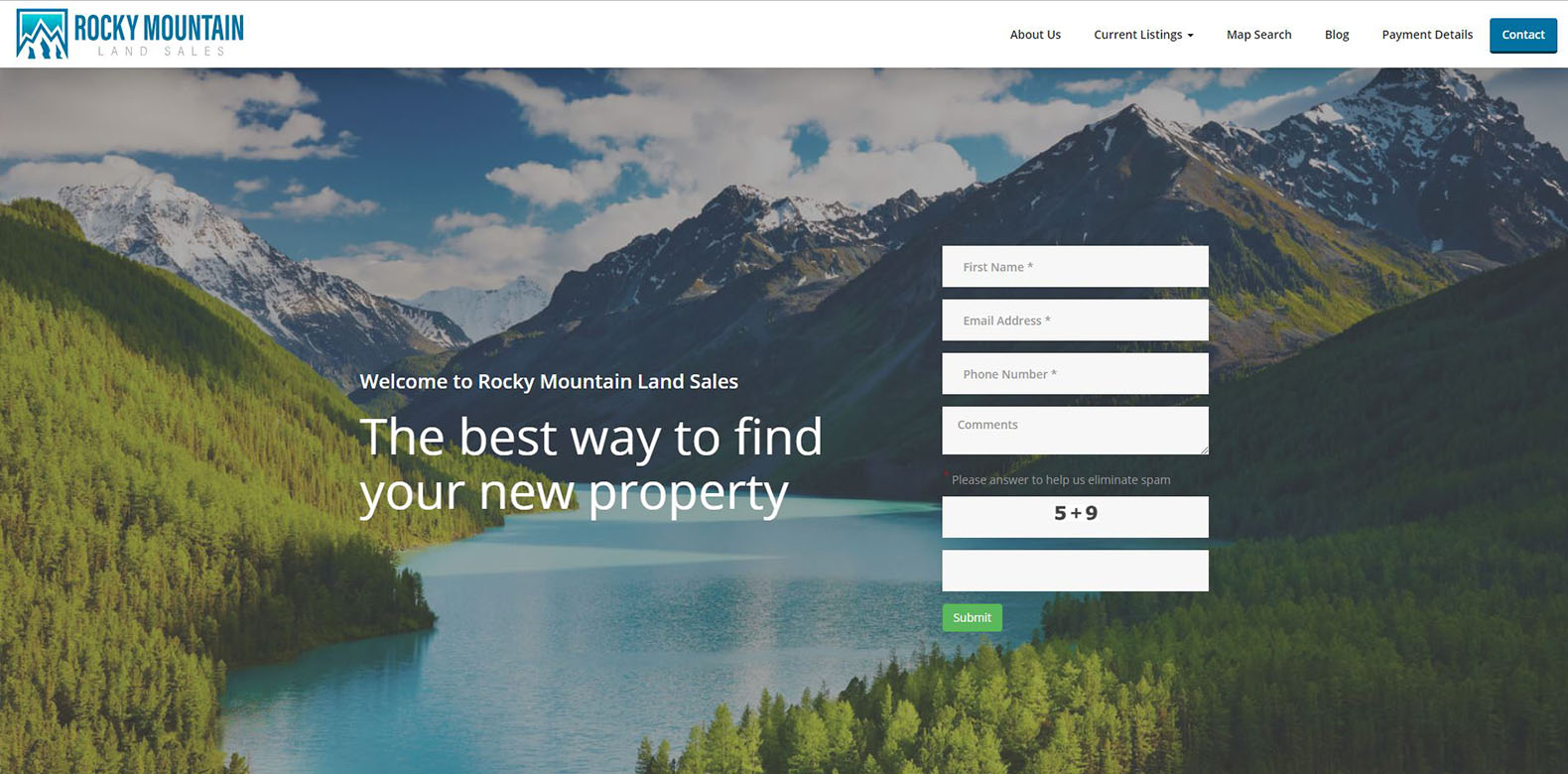The home page of the Rocky Mountain Land Sales website features a clean and organized layout with a mountain-themed aesthetic. 

At the upper left corner, the site branding is displayed in blue against a white background, reading "Rocky Mountain Land Sales." Accompanying this text is a small, blue mountain icon. 

On the upper right, a navigation menu is presented in dark blue or black lettering, including the options: "About Us," "Current Listings" (with a drop-down arrow), "Map," "Search," "Blog," "Payment Details," and a blue rectangle with white lettering that says "Contact."

Dominating the rest of the page is a striking graphic of a mountain landscape. The image features a range of sharp, rocky mountains with patches of snow, greenery on some slopes, and a light green, tree-covered hill in the foreground. A clear blue sky with scattered white clouds stretches above a tranquil stream or lake located centrally within the scene.

Overlaying this picturesque landscape are bold, white letters that warmly invite visitors with the message: "Welcome to Rocky Mountain Land Sales, the best way to find your new property." 

To the right of this welcoming message, an interactive form is available. The form includes several white rectangles for inputting user information: "First Name" with an asterisk indicating it is required, "Email Address," "Phone Number," and "Comments." To combat spam, there is a prompt with the text "Please Answer to Help Us Eliminate Spam," followed by a bold print math problem, "5.9," and a blank white rectangle for the answer. Below this section is a green rectangle button labeled "Submit."